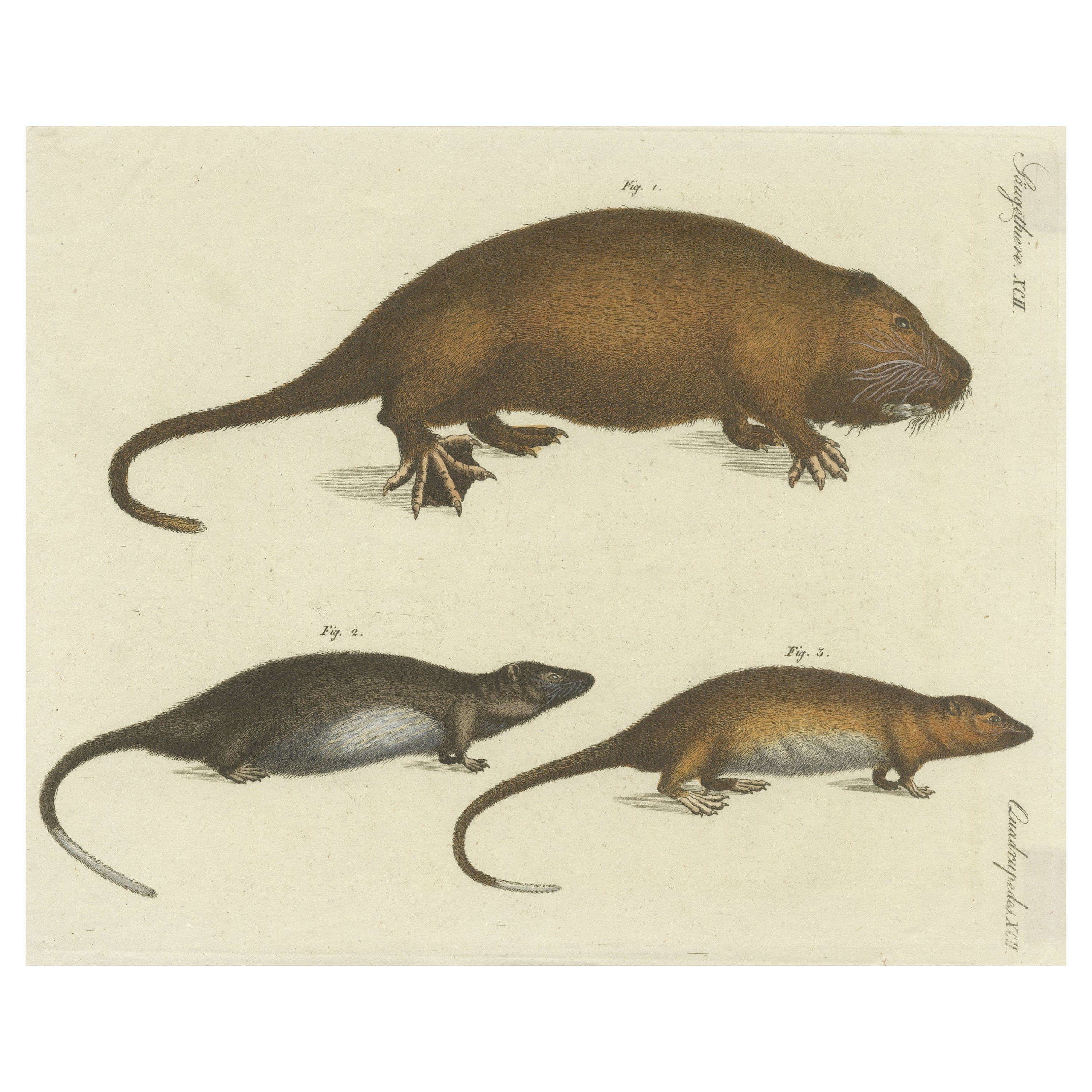The image is a perfectly square drawing with a cream-colored background, featuring three animals arranged in a vertical format. At the top is a large rodent-like mammal, potentially a beaver, depicted with brown fur, a long tail that curls to the left, and prominent black eyes. It has distinct long claws and webbed feet, with whiskers around its mouth. Above this figure is a small label that reads "fig 1." 

Below the top animal, there are two smaller, similarly rendered animals side by side, labeled "fig 2" and "fig 3" respectively. Figure 2 is on the left and has darker fur, nearing black, with a white underbelly. Figure 3, on the right, features brown fur with a lighter tan hue and also has a white underbelly. Unlike the larger animal, these do not have webbed feet, suggesting they may be land dwellers. They are set against the same cream background, indicating an arrangement reminiscent of an old biology textbook or a scientific illustration, possibly emphasizing comparative anatomy among related species.